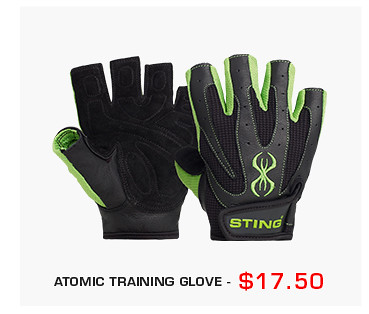The image depicts a pair of black training gloves with lime green trim along the sides and in-between the fingers. The gloves have fingers that are cut off halfway, leaving the fingertips exposed. The palm of the glove can be seen on the left side, completely black in color, while the back of the glove is shown on the right side, featuring some gray stripes. The back of the glove also displays a bright neon yellow or green spider-like insignia. Below this insignia, the word "Sting" is prominently written in fluorescent green with a trademark symbol at the wrist. Along the bottom of the advertisement, it states "Atomic Training Gloves $17.50," with the price written in red.